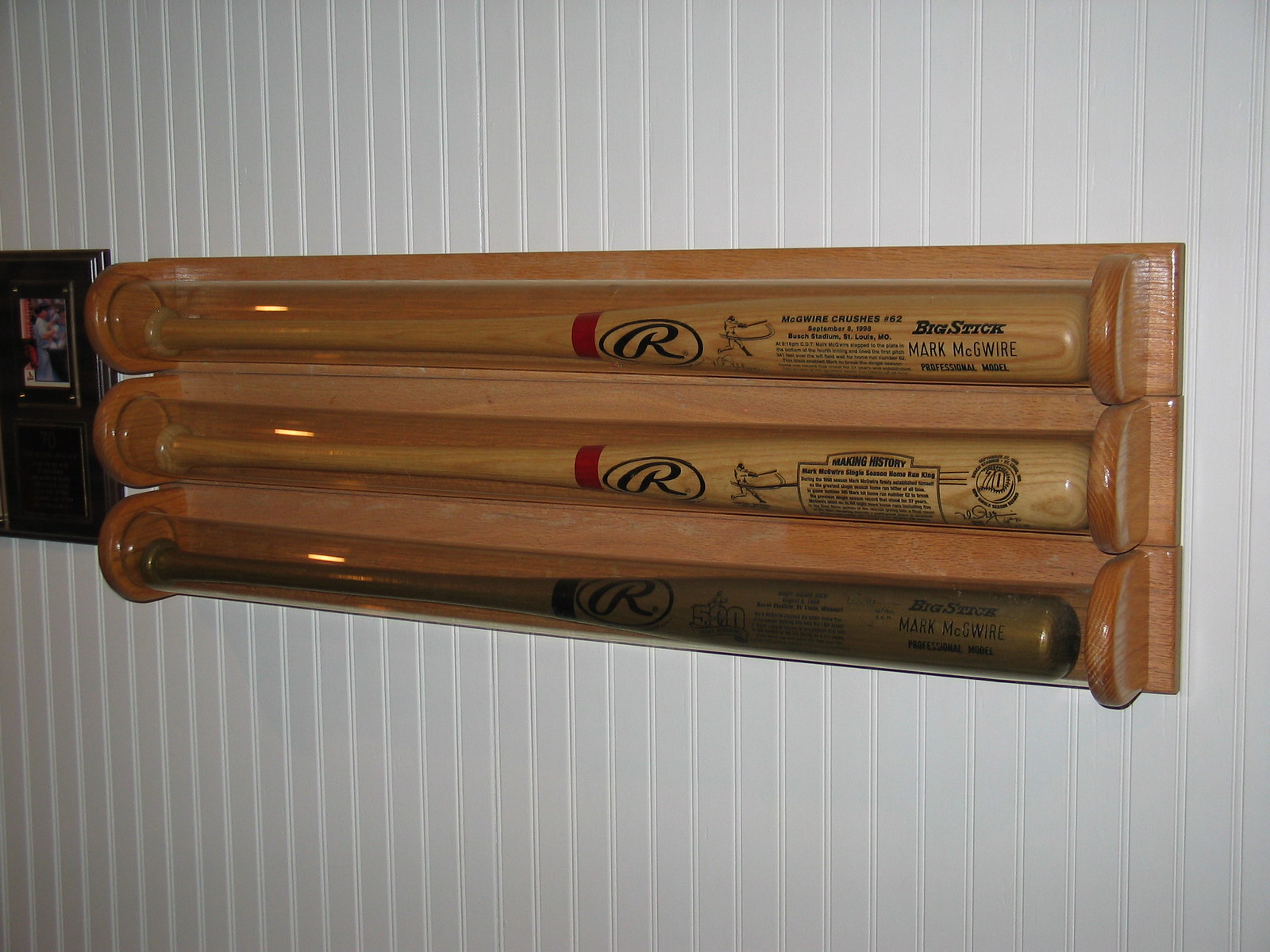This photograph showcases a collector's display of three baseball bats mounted vertically on a white-paneled, wooden wall. The display is a wooden frame with clear glass encasements for each bat. The bats, featuring red bands near the handles and a prominent 'R' logo, are from the 'Big Stick' series and are associated with legendary big league hitter Mark McGuire. The top and bottom bats are lighter in color, with one of them describing McGuire’s iconic "Crushers No. 62" hit at Bush Stadium, St. Louis, Missouri, dated September 8th or 9th, 1993. The middle bat, darker in color, has inscriptions that read "Making History" and "Mark McGuire Professional Model." Despite slight variations in bat color and readability of the text, this curated display eloquently honors McGuire's historic achievements in baseball. Adjacent to the bats is a baseball trading card, further emphasizing the nostalgic and collector's value of the display.